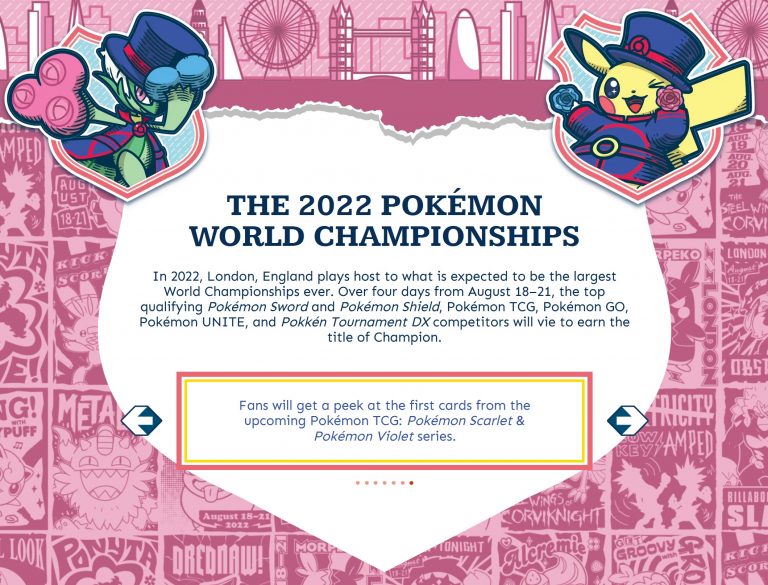This webpage is dedicated to the Pokémon franchise, specifically highlighting the 2022 Pokémon World Championships. Vibrantly adorned with carnival-themed rides at the top border, it features a central banner flanked by two Pokémon characters. The banner prominently announces the 2022 Pokémon World Championships, set to take place in London, England from August 18 to 21. It promises to be the largest championship event ever, spanning four days of intense competition.

Top qualifying champions in Pokémon Sword and Pokémon Shield, Pokémon TCG, Pokémon GO, Pokémon Unite, and Pokkén Tournament DX will vie for the prestigious title. A red-bordered box with a green inner border informs fans that they will get an exclusive preview of the first cards from the upcoming Pokémon TCG: Pokémon Scarlet and Pokémon Violet series.

Navigation arrows on either side of the box allow for page transitions—the left-facing arrow on the left and the right-facing arrow on the right. The webpage indicates that it is the last of seven pages, with the final dot at the bottom highlighted in purple. The entire page is beautifully styled with shades of light, pastel, and darker purple, encapsulating the 2022 Pokémon World Championships theme.